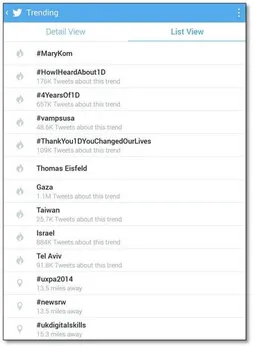This is a detailed screenshot of a Twitter interface, specifically within the "Trending" section. At the very top, there is a light blue header displaying several white icons and text arranged from left to right: a left-pointing arrow, a small bird icon representing Twitter, the word "Trending," and three vertical dots stacked on top of each other located in the top right corner.

Directly below the header, two options are presented on a white background. The "Detail View" option is shown in light gray, indicating it is not currently selected. The "List View" option is displayed in blue and is underlined, signifying that this view is currently active.

Beneath these options, a list of trending terms follows. Each term is accompanied by an icon. The first few entries in the list have a gray flame icon beside them. The detailed trending terms, along with their respective tweet counts, are as follows:

1. **#MaryKom** (spelled as K-O-M)
2. **#HowIHeardAbout1D** – 176k tweets
3. **#FourYearsOf1D** – 657k tweets
4. **#VampsUSA** – 48.6k tweets
5. **#ThankYou1D, You Changed Our Lives** – 109k tweets

Following these, there are additional trending topics without hashtags, such as **ThomasIcefield**.

The screenshot provides a comprehensive snapshot of the trending topics on Twitter at that moment, highlighting user interests and engagement with particular hashtags and terms.